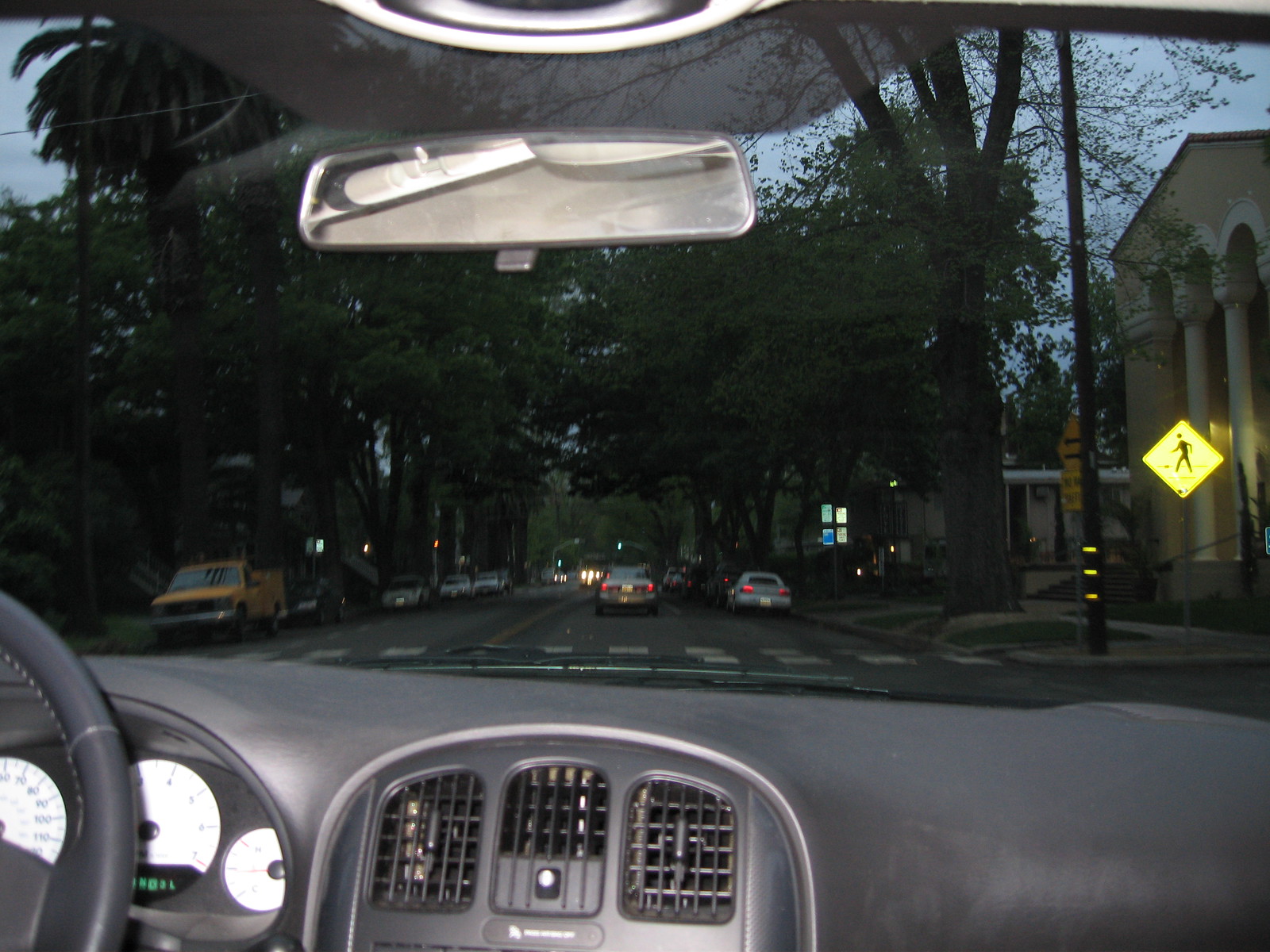The image captures a driver's perspective from inside a vehicle. The dark gray steering wheel is positioned on the left-hand side, partially covering the white-faced speedometer and other instrument gauges on the dashboard, which is also a shade of gray. Below the dashboard, the ventilation system is visible. Through the windshield, a gray road stretches ahead, marked by a central yellow line and a crosswalk. Prominently in the center of the road is a yellow diamond sign featuring a black stick-figure silhouette. 

To the left of the crosswalk, another pole stands with an additional yellow sign. Directly in front of the vehicle is the back of a parked sedan, leading to a line of other cars, including a yellow truck parked on the left side of the road. More vehicles are parked along the right-hand side as well. The scene is framed by leafy green trees and on the far right, the silhouette of a large building with pillars is visible. The rearview mirror above is gray, and a fragment of blue sky peeks through the top of the windshield, adding a touch of brightness to the scene.